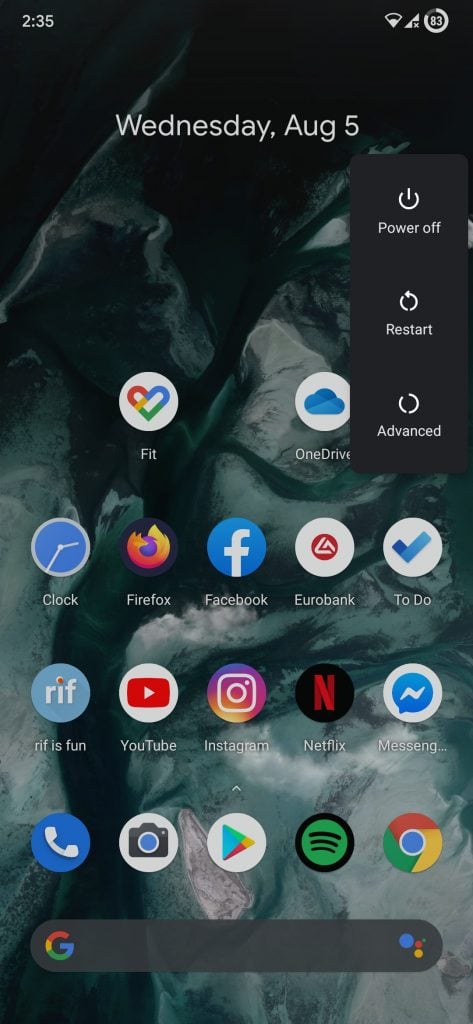**Caption:**

The background of the phone screen displays a serene aerial view of an ocean, showcasing vibrant blue waters interspersed with waves and possibly an island. A noticeable rift runs through the middle, adding depth and intrigue to the scene. The water gradually turns darker, fading to black towards the top of the image.

At the top of the screen, the time is displayed as 2:35, alongside icons for Wi-Fi, data, and a timer indicating 83 seconds. The date is shown as Wednesday, August 5th. A menu on the side offers options to power off, restart, or access advanced settings.

Below this, several app icons are arranged in a grid. The first row includes Google Fit and OneDrive. The second row features the clock, Firefox, Facebook, Eurobank, and To Do apps. The third row lists "Riff is Fun," YouTube, Instagram, Netflix, and Messenger. The fourth row includes essential apps such as the phone app, camera app, Play Store, Spotify, and Google. At the bottom of the screen, a Google search bar is conveniently placed for quick access.